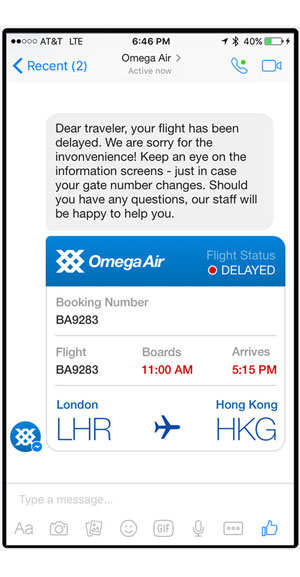This image is a detailed screenshot of a smartphone screen displaying a message from Omega Air. At the very top of the screen, the status bar indicates that the phone is using AT&T as the service provider, the time is 6:46 p.m., and the battery is charged to 40%. Below this, "Omega Air" is prominently displayed in black lettering, with the status "active now" in smaller gray lettering underneath.

On the far left, there is a caret symbol which implies the option to navigate back to a recent messages list, indicated by the text "Recent (2)", suggesting there are two recent messages.

In the center of the screen, a message from Omega Air reads: "Dear Traveler, your flight has been delayed. We are sorry for the inconvenience. Keep an eye on the information screens, just in case your gate number changes. Should you have any questions, our staff will be happy to help you."

Below the message is a blue box containing the Omega Air logo and the words "Omega Air." It also highlights the flight status with the word "Delayed" accompanied by a small red circle. Further details provided include the booking number and flight number, both listed as BA9283. The flight details indicate boarding at 11 a.m. and arrival at 5:15 p.m. The origin is London Heathrow (LHR), and the destination is Hong Kong (HKG).